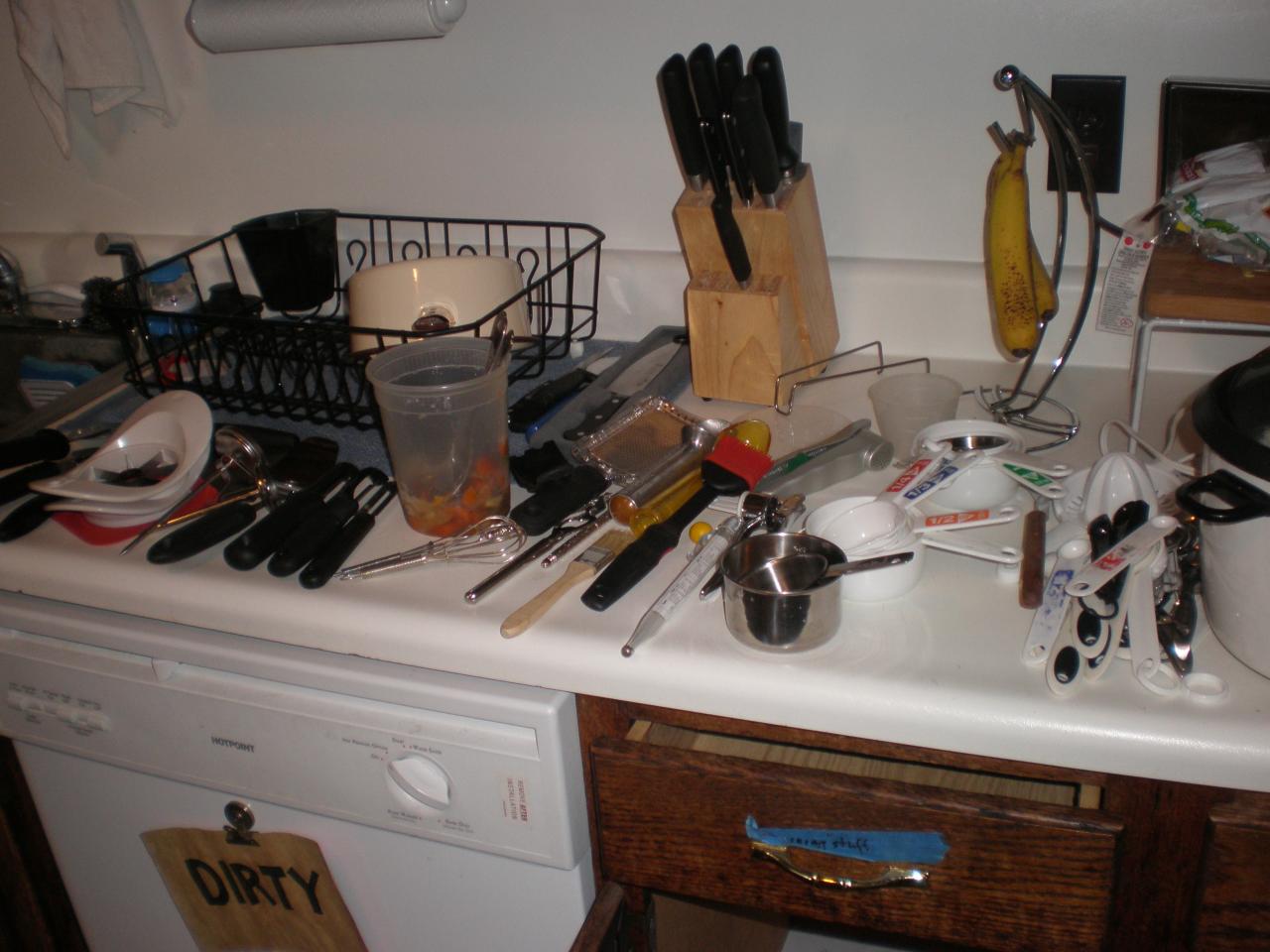A photograph captures a somewhat dimly lit kitchen, highlighting a cluttered white countertop against a backdrop of white walls. In the upper left corner, a stainless steel sink partially appears, complete with a sprayer fixture. Adjacent to the sink is a black dish drying rack holding a beige pot, alongside an assortment of oddly shaped white bowls. In the midst of the kitchen chaos, two black-handled vegetable peelers lie nearby.

Positioned right of the dish rack sits a large, lidless plastic container, akin to those from a Chinese take-out restaurant, containing two silver-topped utensils. In front of this container, a small silver whisk rests on the countertop. Shifting right, a paintbrush with a light brown handle appears amidst what seems to be the contents of a toolkit, possibly including the edge of a wrench. Next to these tools are two silver measuring scoops.

Leaning against the white backsplash, a butcher block knife holder stands tall, accommodating approximately eight knives, each with a black handle. To its right, a chrome banana holder supports two ripened bananas. The lower right section of the countertop displays more kitchen utensils, including white plastic measuring spoons and a manual white plastic orange juicer.

Below the countertop is a dishwasher adorned with a magnet. Attached to the magnet, a brown paper bag prominently features the word "dirty" written in black marker, summarizing the overall cluttered yet intriguing scene of the kitchen.